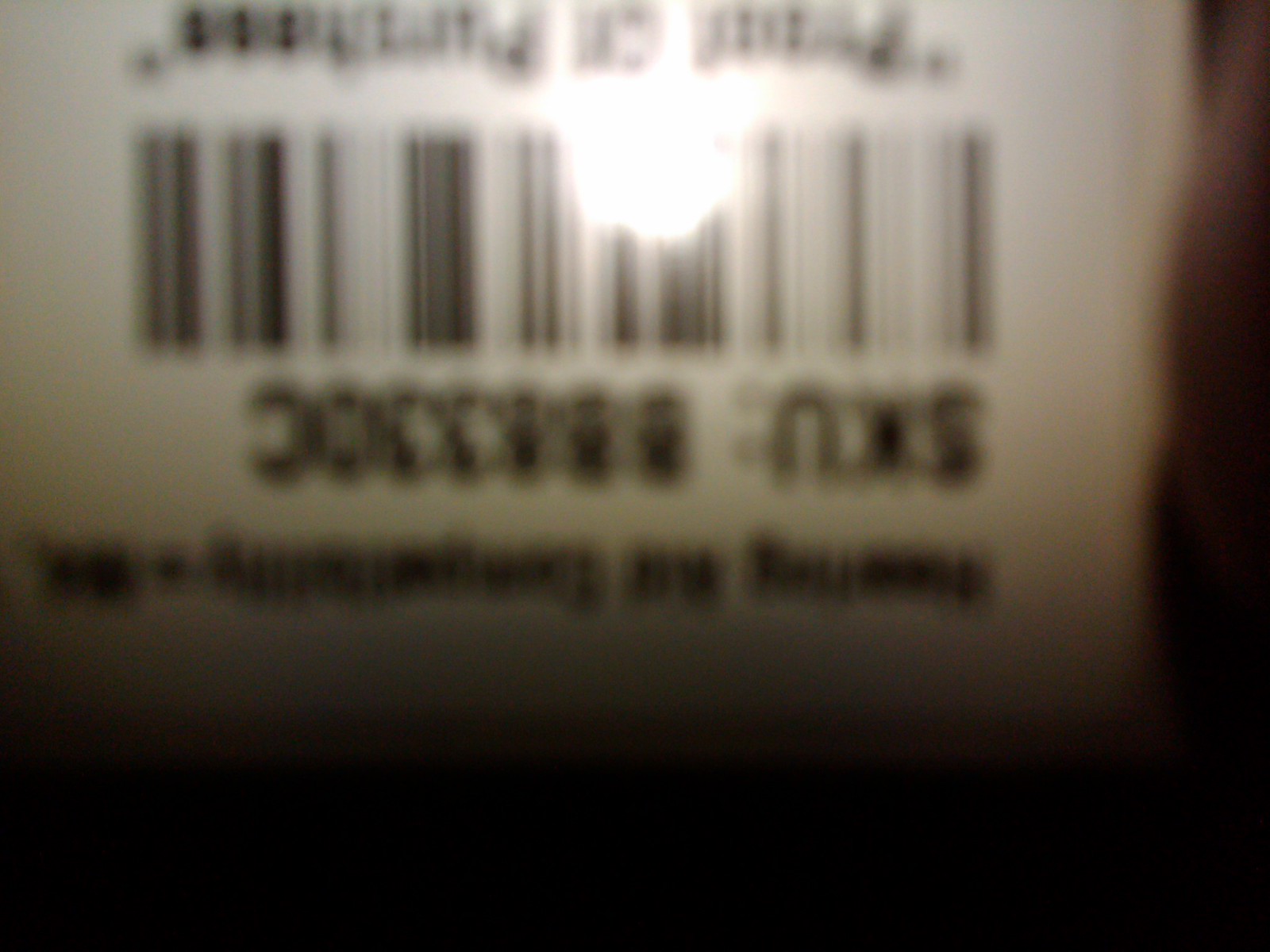The image depicts a blurry and distorted UPC code that is both upside down and backwards, making it difficult to decipher. A line of text is positioned approximately halfway up the image, which would be located directly beneath the UPC code if the image were oriented correctly. However, the text is too blurred to be legible, and words such as "healing" and "ability" are barely discernible. Above this line of text is the UPC code itself, which is similarly obscured by the poor image quality. At the very top of the image, there is additional text, but it remains unreadable due to the same blurriness.